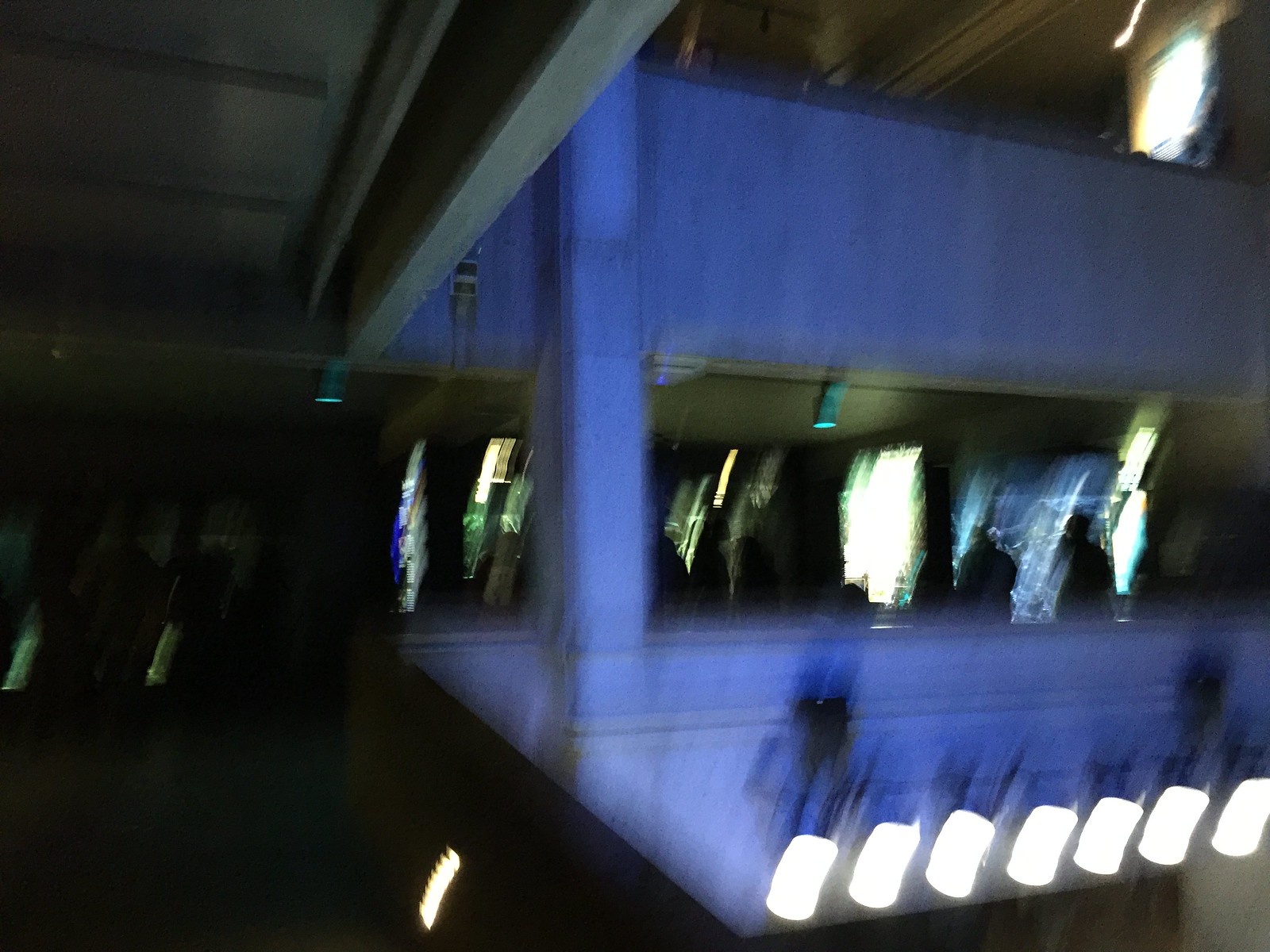In this extremely blurry nighttime photograph taken in a dimly lit environment, the setting appears to be a multi-story lounge, nightclub, or bar. The image reveals a lower floor with a second story above it. The scene is dominated by blue lighting or possibly a blue structure that's illuminated, creating a striking contrast against the surrounding darkness. The left side of the image remains significantly darker, with minimal lighting illuminating the interior. A row of white cylindrical lights can be seen at the bottom right, adding to the eclectic illumination. The photo captures the vague silhouettes of people standing around, suggesting a bustling atmosphere akin to a party or social gathering. Vending machines are also noticeable on the photographer’s level, implying that guests might be grabbing snacks or drinks. Despite the poor quality and the camera shake, the photograph provides a glimpse into a lively and complex, possibly cement-structured, space.